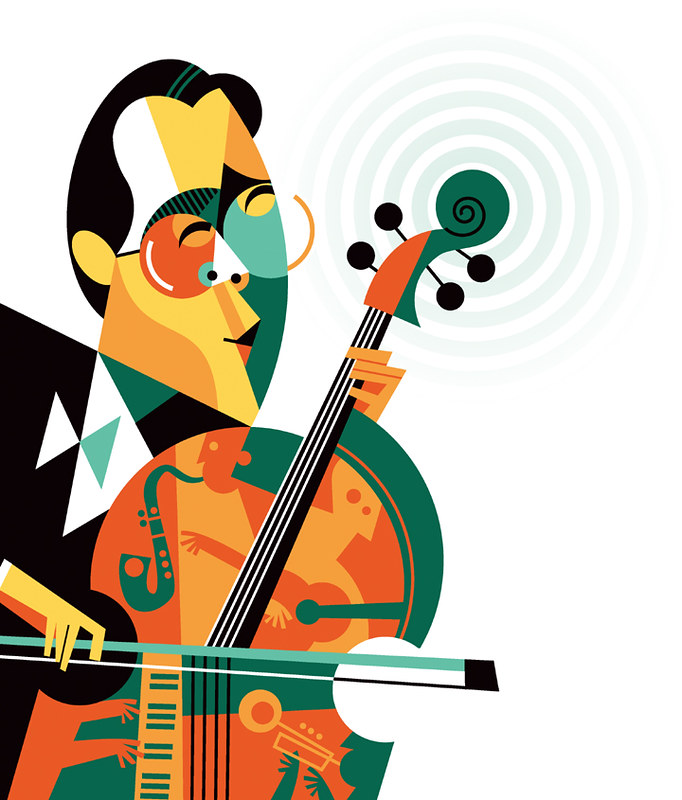In this highly stylized, cubist-inspired drawing—reminiscent of illustrations you might find in The New Yorker—a male musician, resembling Yo-Yo Ma, is playing a cello. The angular yet curvilinear lines capture his figure emerging from the left of the image. The musician, depicted with glasses and black hair, is clad in a black and white tuxedo with hints of green. The cello itself stands out vividly with green and orange hues. Adding to the composition, there's an intricate circle and spiral design in the top right corner. The drawing, characterized by shades of green, red, yellow, orange, black, silver, gray, and white, presents a compelling blend of geometric abstraction and vibrant color, translating the essence of a musical performance into visual form. The musician is holding a bow in his right hand while looking towards the right. Although it's difficult to ascertain whether he's standing or sitting due to the cropped nature of the image, the artwork communicates an ethereal quality, leaving the setting ambiguous.